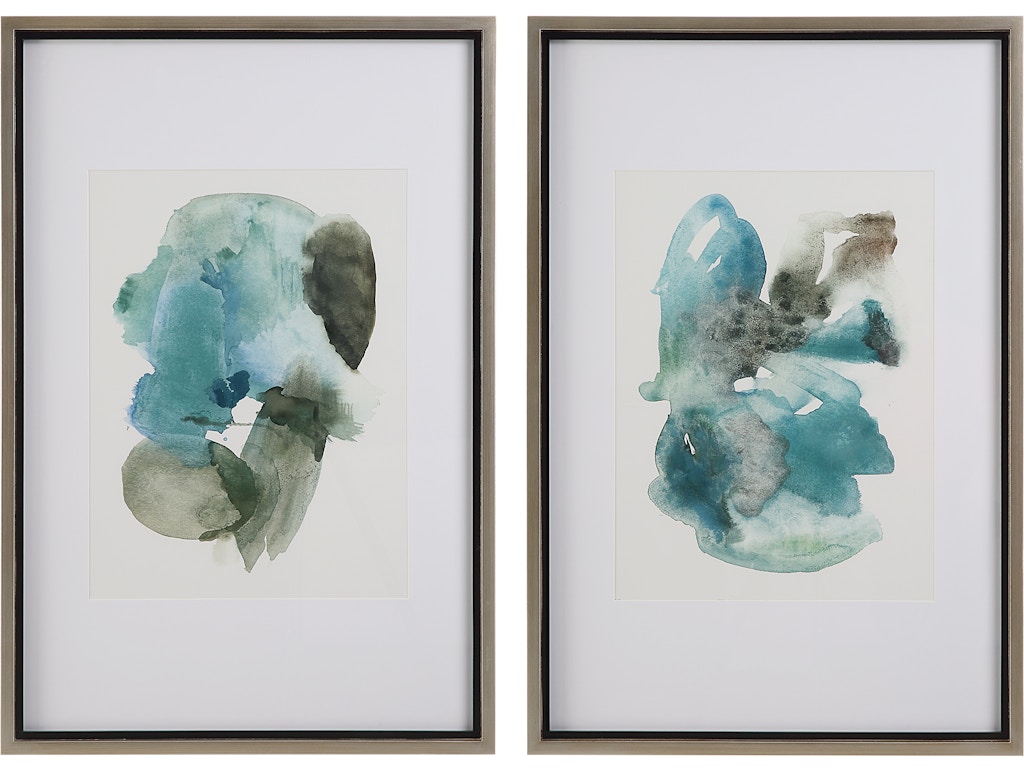The image features two art prints displayed side by side, each enclosed within a multi-layered frame. The outermost frame is a combination of light blue and light brown, bordered on the inside by a darker black frame. Inside this is another inner frame made of white cardboard or paper. At the very center are the actual paintings themselves, characterized by a light gray background.

The artworks appear as abstract watercolor compositions in shades of blue, gray, and brown. The forms are amorphous and evoke a sense of fluidity, reminiscent of clouds or possibly even aquatic elements like fish or coral. The overall aesthetic is subtle and open to interpretation, with the shapes being splotched together in a way that suggests a natural, underwater world, yet remains vague and non-descript. The combination of colors and abstract forms gives a soothing, almost oceanic feel to the prints.